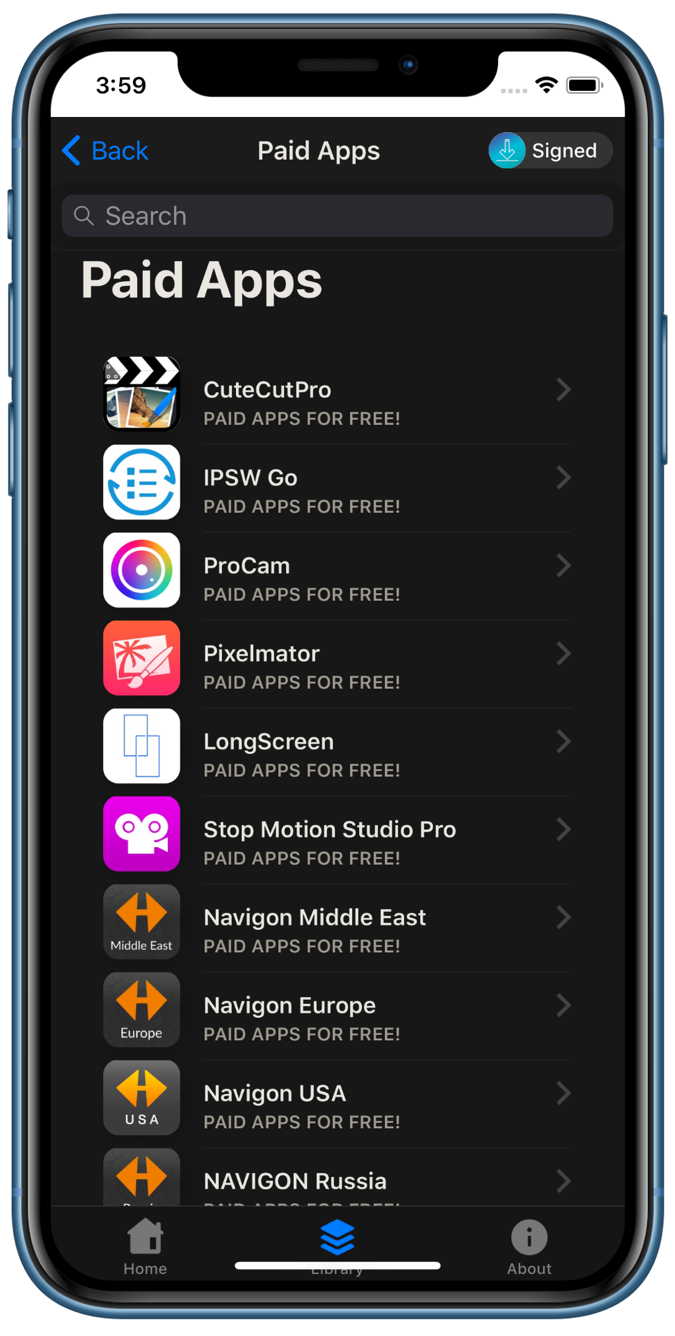The image displays a smartphone with a blue-colored interface. The screen shows the time as 3:59, alongside icons indicating a Wi-Fi connection, full battery, and a 'back' hyperlink symbolized by a blue less-than symbol. At the top, there's an empty search bar, and immediately below it, in large white letters, is the heading "Paid Apps."

Beneath the heading, the list begins with "CuteCut Pro" and continues with several other apps: IPSW Go, ProCam, PixelMaster, LongScreen, StopMotionStudio Pro, Navigon Middle East, Navigon Europe, Navigon USA, and Navigon Russia. Each app name is followed by the text "paid apps for free" and is accompanied by a unique icon on the left side and a greater-than symbol on the far right, indicating the option to navigate further into each app's details.